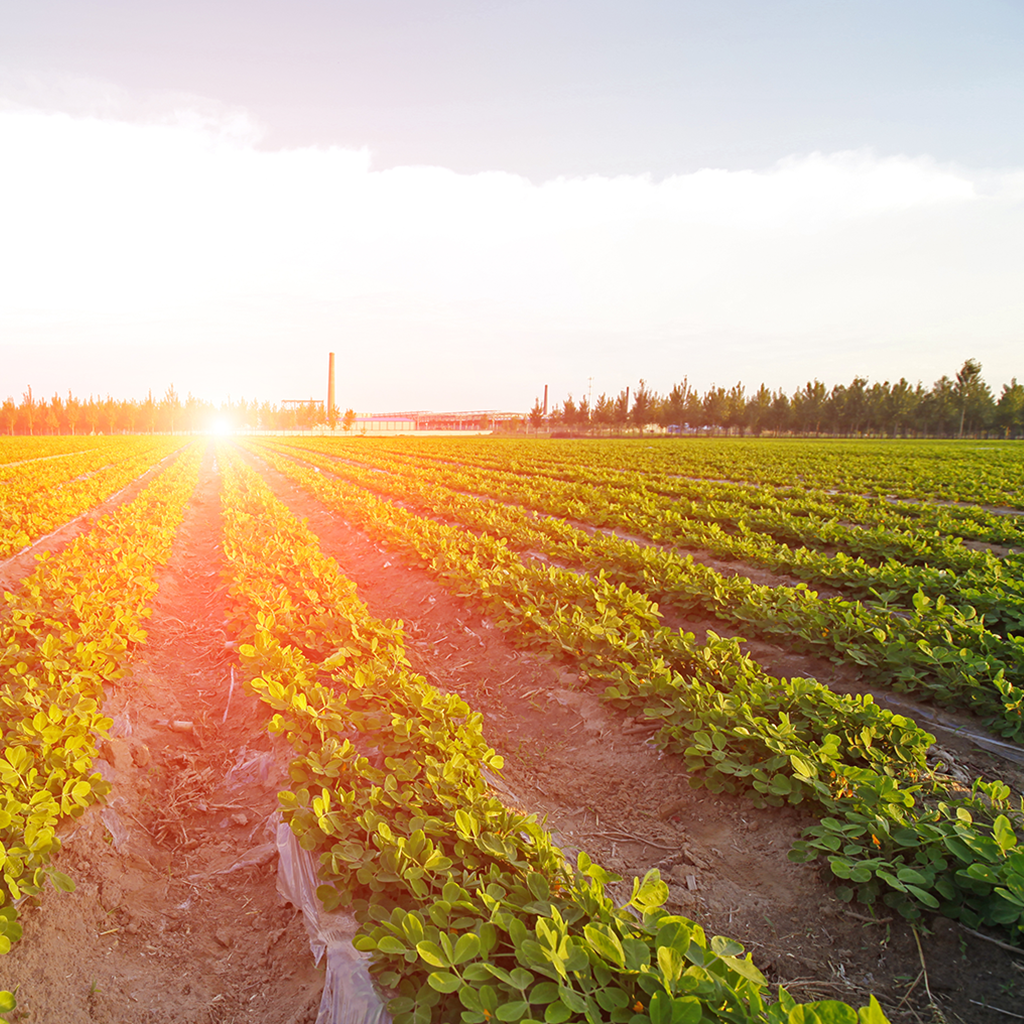The photograph captures a vast and orderly farm with rows upon rows of vibrant green crops, each neatly divided by strips of soil resembling small ditches. The green crops, possibly strawberry plants given their low green stems and rounded foliage, dominate the forefront of the image. In the lower right-hand corner, we get a close-up view of these lush plants. The systematic rows lead the eye towards the horizon, where the sun is either setting or casting a bright light towards the far end of the middle row, illuminating some farm equipment. Surrounding the farm are several rows of trees that frame the background. Towards the left side of the horizon, there is a prominent stack or smokestack, while to its right stands a silo and a building. Above these elements, the sky transitions from grey to a mix of white cloud and soft blue. The entire image is presented in a square format, encapsulating the serene yet industrious farm scene.